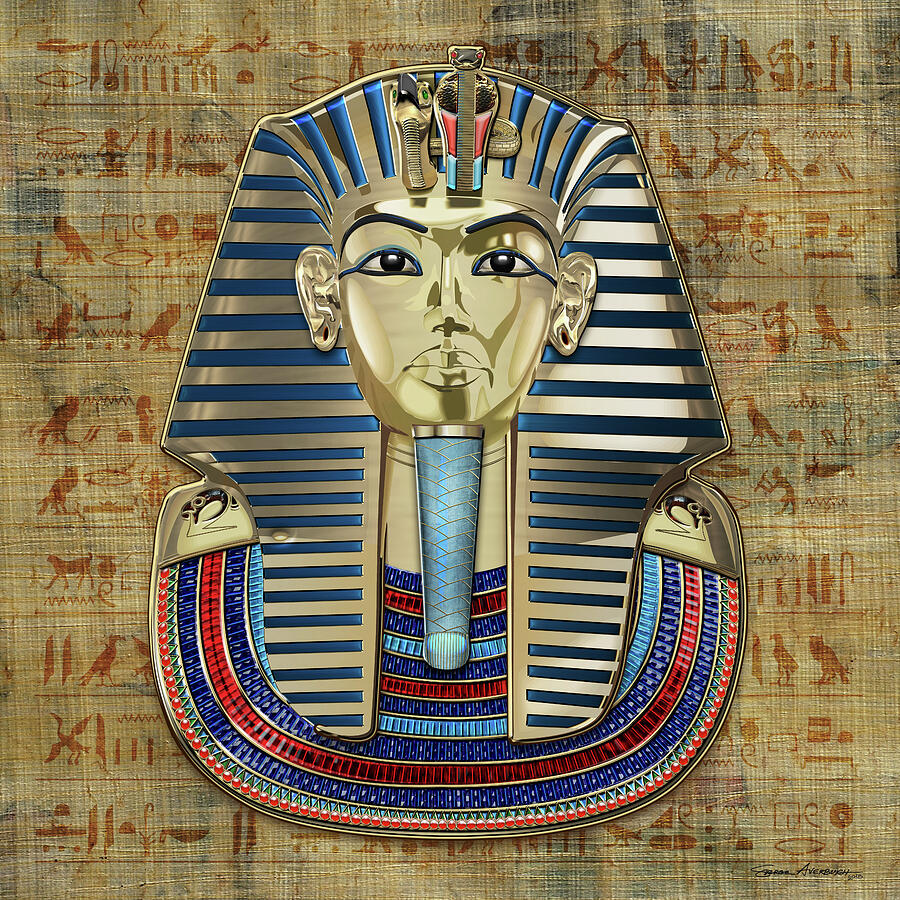The image is a digitally generated illustration of Tutankhamen's iconic gold death mask. The mask itself is meticulously detailed with an intricately painted gold face, adorned with a prominent blue braided beard. The headdress is dominated by alternating blue and gold stripes and is further embellished with dual motifs of a snake and a bird at the forehead. The eyes are outlined in a striking blue eyeliner, offering a lifelike gaze. The mask's necklace features a pattern of alternating colors: light blue, dark blue, and red, set in a repeated sequence. The backdrop of the image simulates a papyrus or linen material, adorned with red and brown hieroglyphics that lend an authentic ancient Egyptian aesthetic. Overall, the image is rendered in a square format, with the visually rich mask at the center, surrounded by the textural background, capturing the essence and grandeur of the pharaoh's burial art.